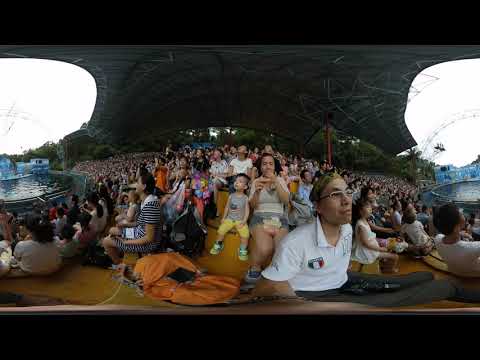The image portrays a large, excited crowd seated in an outdoor auditorium, suggesting a mild, clear day given the abundance of casual attire like shorts and t-shirts. The auditorium envelops the scene in a panoramic 360-degree, or possibly 180-degree, fisheye view creating a somewhat disorienting, yet immersive, perspective. 

The audience, including men, women, and children of varying ages and likely South Asian descent, all bear expressions of anticipation, particularly a man in a white polo shirt adorned with an Italian flag-colored logo, who stands out clearly in the foreground.

In the distance, to both the left and right, are bright blue pools of water with noticeable ripples, hinting at an upcoming aquatic show possibly featuring dolphins or killer whales given the large pool's setup. The setting, which might evoke an open-air cave or tunnel with beams of white light illuminating sections of the crowd, keeps them captivated and collectively engaged as they await the spectacle to unfold.